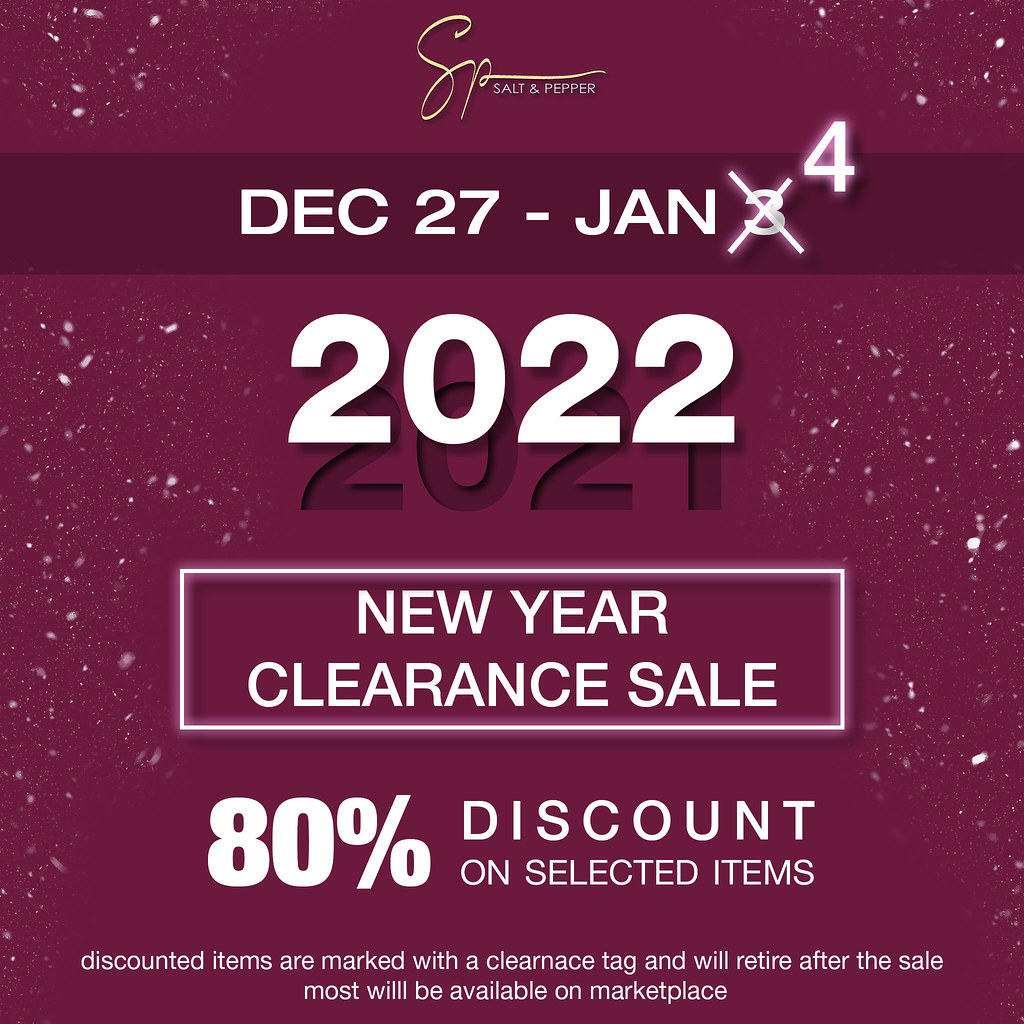This advertisement for S&P Salt and Pepper prominently features a large purple background with white text. At the very top center, the company's logo is displayed with an "S" and "P" in cursive, connected, followed by "Salt and Pepper" in small white text. Directly below, there's a dark purple line with "December 27 - Jan" in white text, but the "3" is crossed out and replaced with a "4" in the upper right corner, indicating an extension of the sale to January 4th. Below this, the year "2022" is displayed, shadowed by a lighter "2021" in the background, symbolizing the transition to the new year. Further down, a white-text square reads "New Year Clearance Sale," and outside the square, there's an "80% discount on selected items" announcement. At the bottom, it notes that discounted items are marked with a clearance tag and will retire after the sale, though most will be available on Marketplace. The background also features white and pink speckles on the left and right, resembling falling snow.